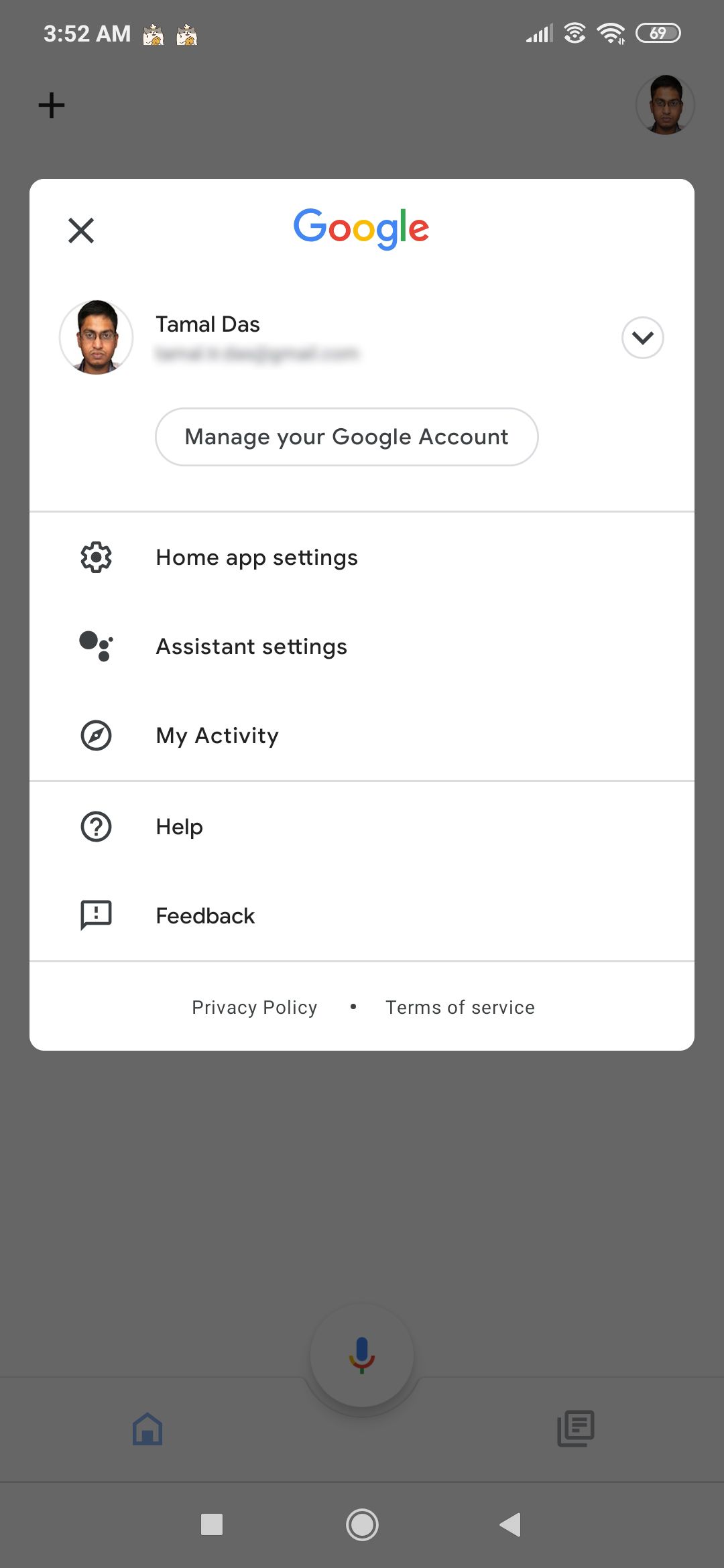This image is a screenshot from a mobile Android device, identifiable by the three navigation buttons at the bottom: a square, circle, and back arrow. The background is dim and somewhat obscured by a prominent white pop-up from Google that dominates most of the screen. This pop-up is a large white rectangle featuring the Google logo at the top, displaying its characteristic colors: green, red, yellow, and blue in a repeated sequence.

Beneath the logo is the user's name, "Tarnal Das," accompanied by a profile picture on the left side. The user's email account is blurred out for privacy. Directly below this information is a clickable bubble labeled "Manage your Google account."

Further down, there is a series of icons with labels:
1. A gear icon labeled "Home app settings."
2. The Google Assistant icon labeled "Assistant settings."
3. A compass-like icon labeled "My activity."
4. Additional buttons for "Help" and "Feedback" are also visible.

The screenshot effectively captures the Google account management interface on an Android device, detailing various settings options available to the user.